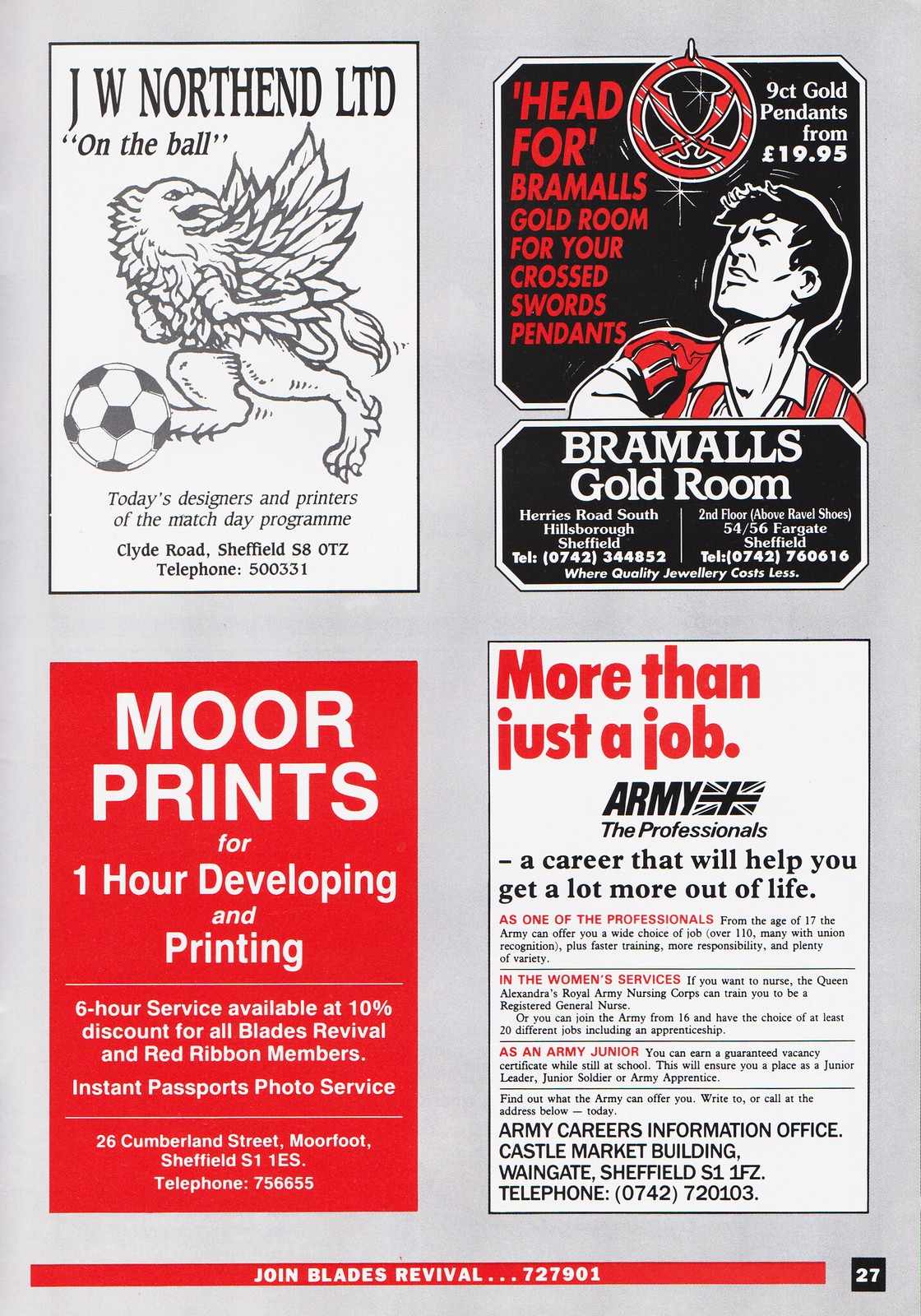The image is a scan of a magazine page divided into four rectangular advertisements, set against a light gray background. At the top left, there's an ad for JW North End Ltd., showing a griffin kicking a soccer ball, complete with the company's address and phone number. Adjacent to it on the upper right, is an ad for Brommel's Gold Room, featuring a swashbuckling prince, promoting their nine-karat gold Crossed Sword Pendants, also including contact details. The bottom left rectangle features an ad for More Prints, offering one-hour developing and printing services, along with the address, phone number, and additional discounts for Blades Revival and Red Ribbon members. Lastly, the bottom right box showcases an advertisement for the British Army Career Center, emphasizing the slogan "More Than Just a Job" and assuring a rewarding career. The bottom of the page has a strip urging readers to "Join Blades Revival" with a provided phone number, and the page is marked as number 27 in the bottom right corner.